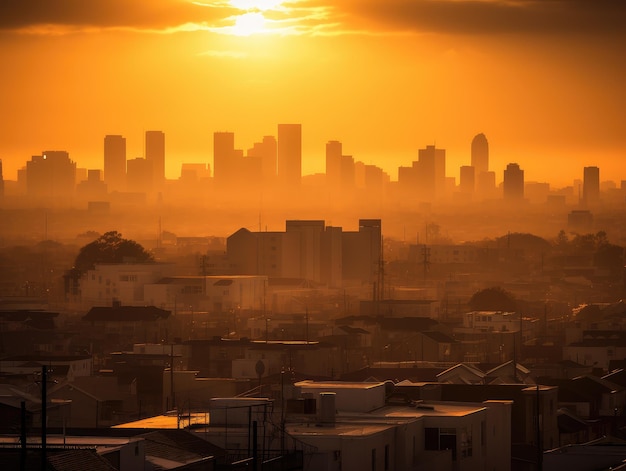The image captures a foreign cityscape near sunrise or sunset, bathed in a hazy orange and yellow glow with the sun peeking through some clouds near the top of the picture, casting shafts of light and contributing to the scene's warm palette. The backdrop features silhouettes of tall, backlit skyscrapers, while smaller, white, basic square-like buildings and possibly worn-down residential or commercial structures are seen in the foreground. A slight mist or fog, potentially early morning dew or smog, hovers over the city, adding to the hazy ambiance. Scattered trees, telephone lines, and power lines further detail the scene, enhancing the sense of an urban environment transitioning through the calm, transitional time of day.